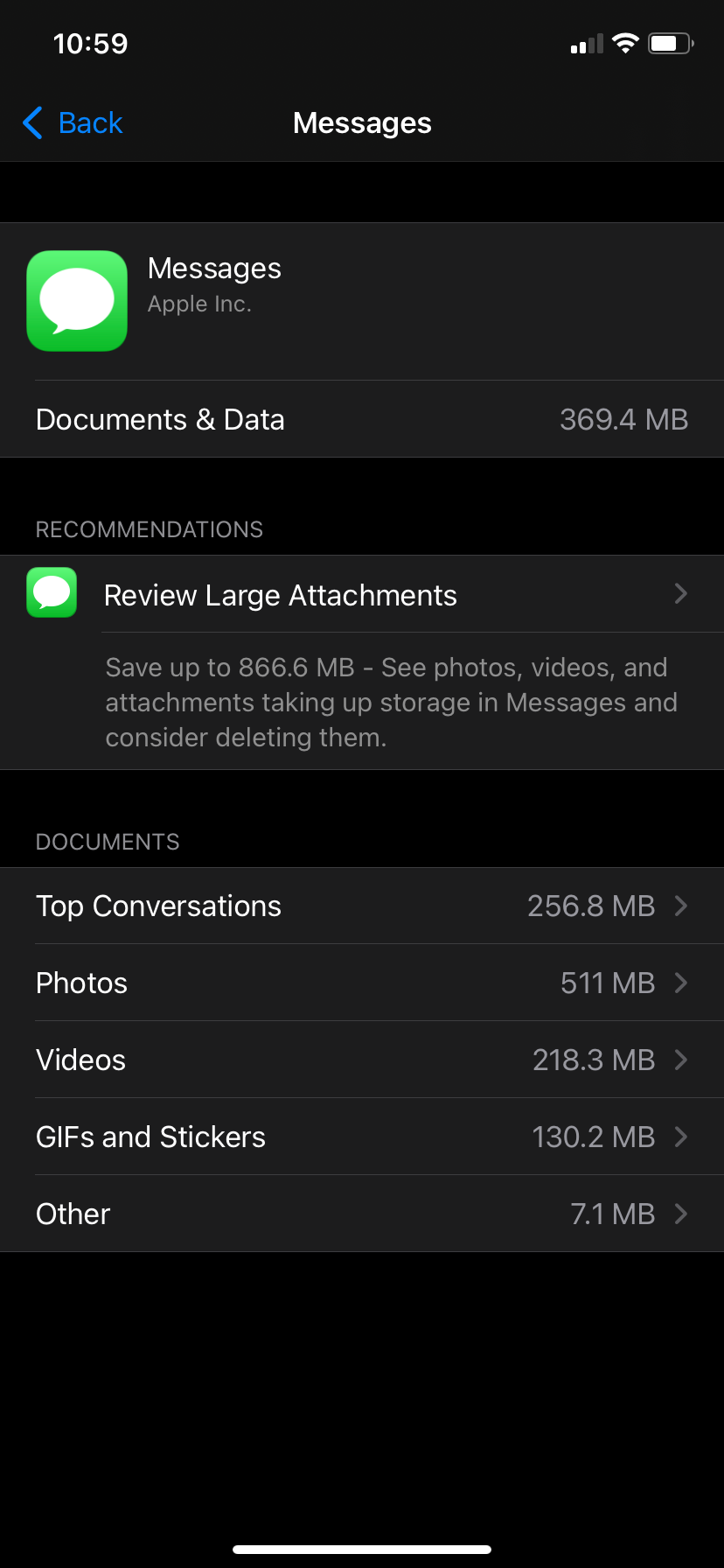In this image of an iPhone screen displaying the settings area for messages, the background is black. At the top left corner, the time is shown as "10:59" in white text. On the top right, there are various connectivity indicators including carrier signal, Wi-Fi, and battery life. Below the status bar, a blue "Back" button with an arrow is visible, and next to it, in white text, is the word "Messages."

The central part of the screen prominently features the messaging icon—a green square with a white speech bubble. Below this, the text "Messages, Apple Inc." is displayed, followed by "Documents & Data," showing a storage usage of "369.4 MB."

Under the "Documents & Data" section, the "Recommendations" area is highlighted. It suggests that users review large attachments to save up to "866.6 MB." The green messaging icon with the white speech bubble reappears here. If selected, this option allows users to manage their storage by reviewing and potentially deleting photos, videos, and attachments taking up space.

Further down, the "Top Conversations" section lists various data categories, indicating their respective storage usage: "Documents" at "256.8 MB," "Photos" at "511 MB," "Videos" at "218.3 MB," "GIFs and Stickers" at "130.2 MB," and "Other" at "7.1 MB."